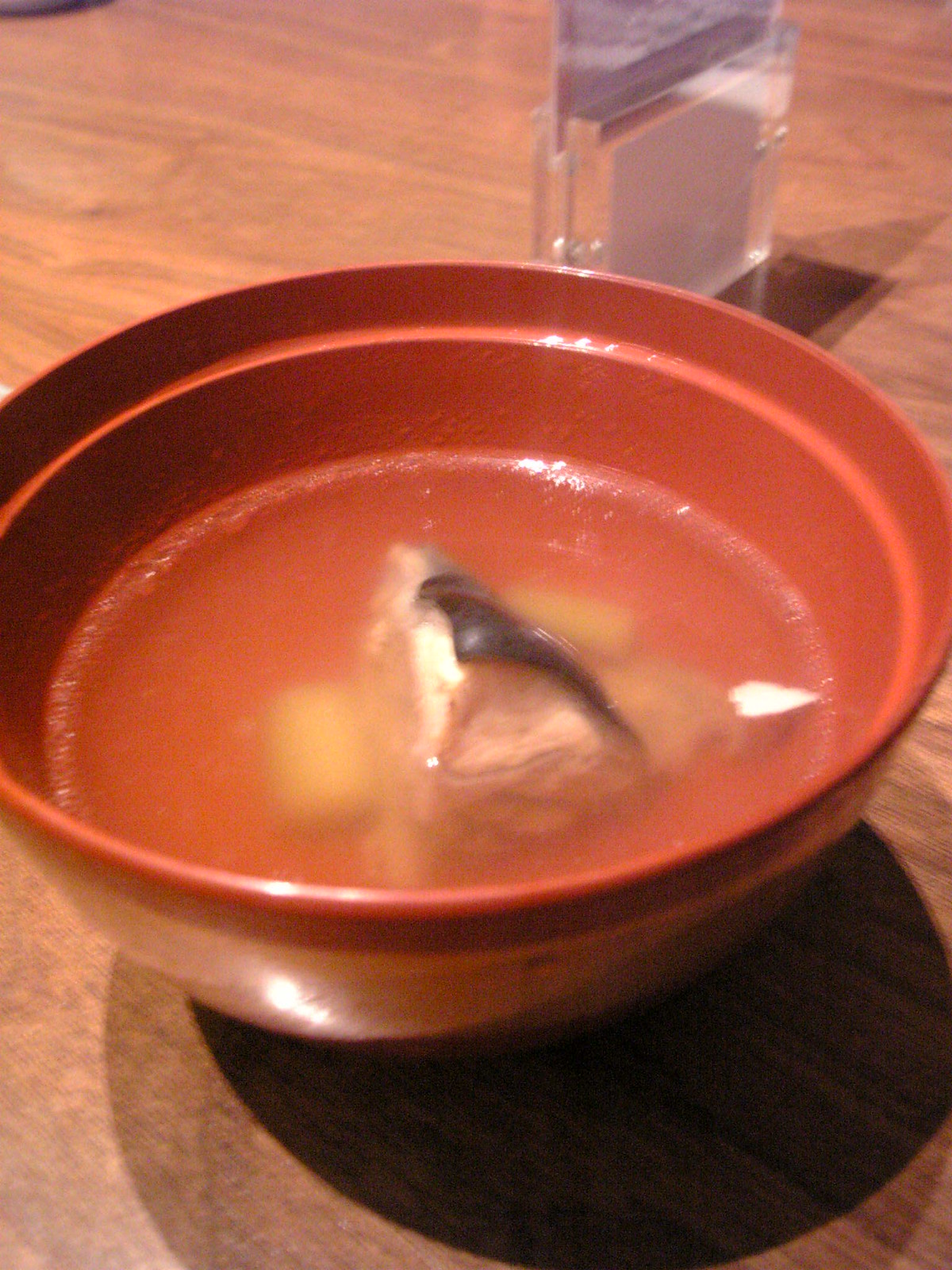A richly detailed image showcases a vibrant, dark red bowl filled with a creamy, white broth. Suspended in the broth is a piece of meat, likely a tender cut of chicken or pork, though its visibility is somewhat obscured, giving an air of mystery to its true identity. Also nestled within the soup are light-colored vegetables, adding texture and contrast to the dish. The surface of the broth displays a delicate glisten of oil, indicating a flavorful, slow-cooked preparation. The bowl is set on a rustic wooden table, contributing a cozy, homely ambiance to the scene. Partially visible in the cropped frame, there appears to be a glass, hinting at a complementary beverage just out of sight.